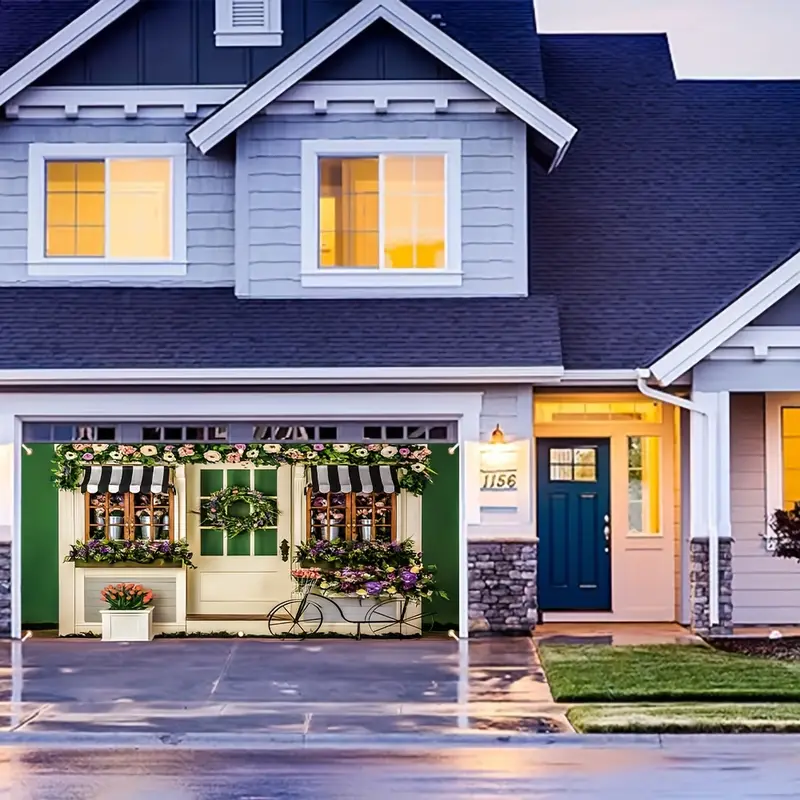This photo captures the front of a modern, two-story, upper-middle-class home at 1156. The house is clad in blue vinyl sidings with a dark blue roof and features eaves with windows on the second floor. The recessed entryway, supported by columns with cobblestone brick bases and topped with white paneling, features a blue front door.

The garage door, unlike typical designs, is open and painted to resemble the entrance to a quaint flower shop. It features detailed flower beds, a wreath, and decorative milk cans, lending it a boutique-like charm. Inside, the garage is filled with various plants and flowers, creating the illusion of a nursery. A bicycle, adorned with plants, leans against the side, enhancing the rustic appeal. Additionally, a separate plant pot with pink flowers is placed to the left.

The image appears to be taken in the evening, with lights visible on the second floor, adding warmth to the scene. The concrete driveway and the damp road and sidewalk indicate recent rainfall, adding a fresh and reflective quality to the setting. The overall ambiance suggests that the garage is transformed into a green haven, possibly used for photoshoots or recordings, making this home uniquely picturesque.